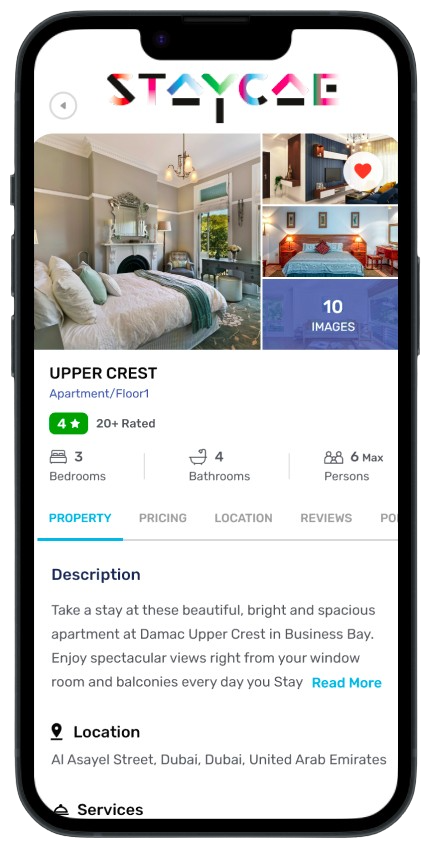This image captures a mobile phone screen displaying a listing for a luxury apartment. The top of the screen features the stylized text "STAY-K," spelled out in ornate lettering that makes the exact spelling somewhat ambiguous, resembling "S-T-A-Y-C-A-E." 

The main content shows several photos, including a beautifully decorated bedroom that exudes elegance and comfort, accompanied by two additional images depicting other rooms within the residence. 

Beneath the photographs, there is a detailed listing header that reads: "Upper Crest Apartment / Floor 1," marked with a four-star rating and noted to have over 20 reviews. The property boasts three bedrooms, four bathrooms, and a maximum occupancy of six people. 

Further down, the description entices potential guests with promises of bright and spacious accommodations at the Damac Upper Crest in Business Bay. Guests are invited to enjoy stunning views from the windows, rooms, and balconies throughout their stay. The listing also includes options to view more details about pricing, location, reviews, and services, along with a "Read More" link for an extended description.